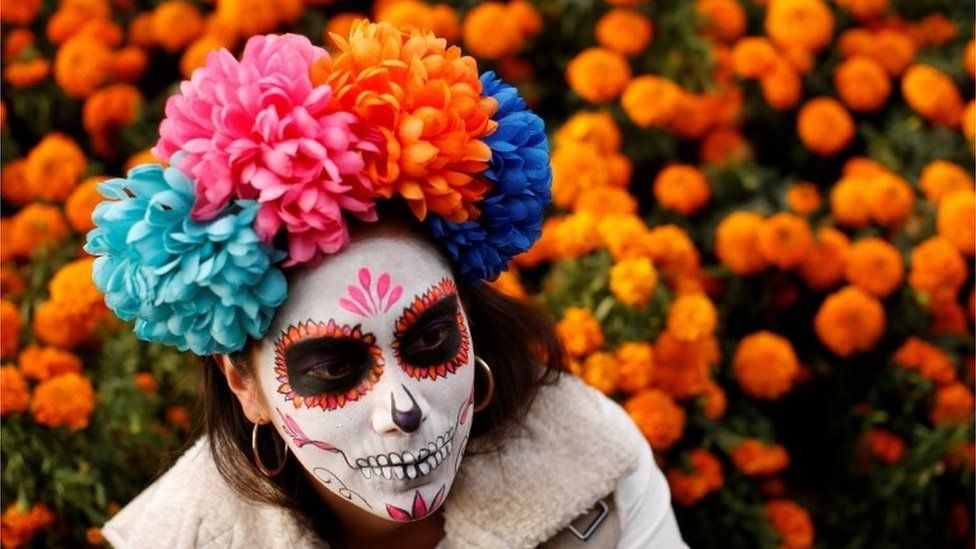In this vibrant and intricate image, a woman adorned in elaborate Dia de los Muertos (Day of the Dead) face paint captures the viewer's attention. She has short dark brown hair, accentuated by a headband of vivid flowers in hues of turquoise, pink, orange, and blue. Her face is completely painted white, with distinctive black paint around her eyes, giving her a skeletal visage. The eyes are adorned with orange flower petals, while her nose is painted black to simulate a skull's nose cavity. Her mouth is crafted into a skeletal grin, with white teeth outlined in black extending across her lips.

Intricately detailed pink flowers are painted on her forehead, cheeks, and chin, accompanied by squiggly lines that enhance the skull illusion. She wears two large hoop earrings and is captured gazing off to the side, projecting a haunting, serene demeanor. She dons a fur-collared coat over a white shirt, adding a textural contrast to the vivid face paint and the bright floral elements.

In the background, an abundance of rich orange flowers, likely carnations, with lush green leaves, creates a natural, vivid backdrop that complements her floral headband. The overall composition exudes a mix of melancholy and beauty, blending the themes of life and death seamlessly.